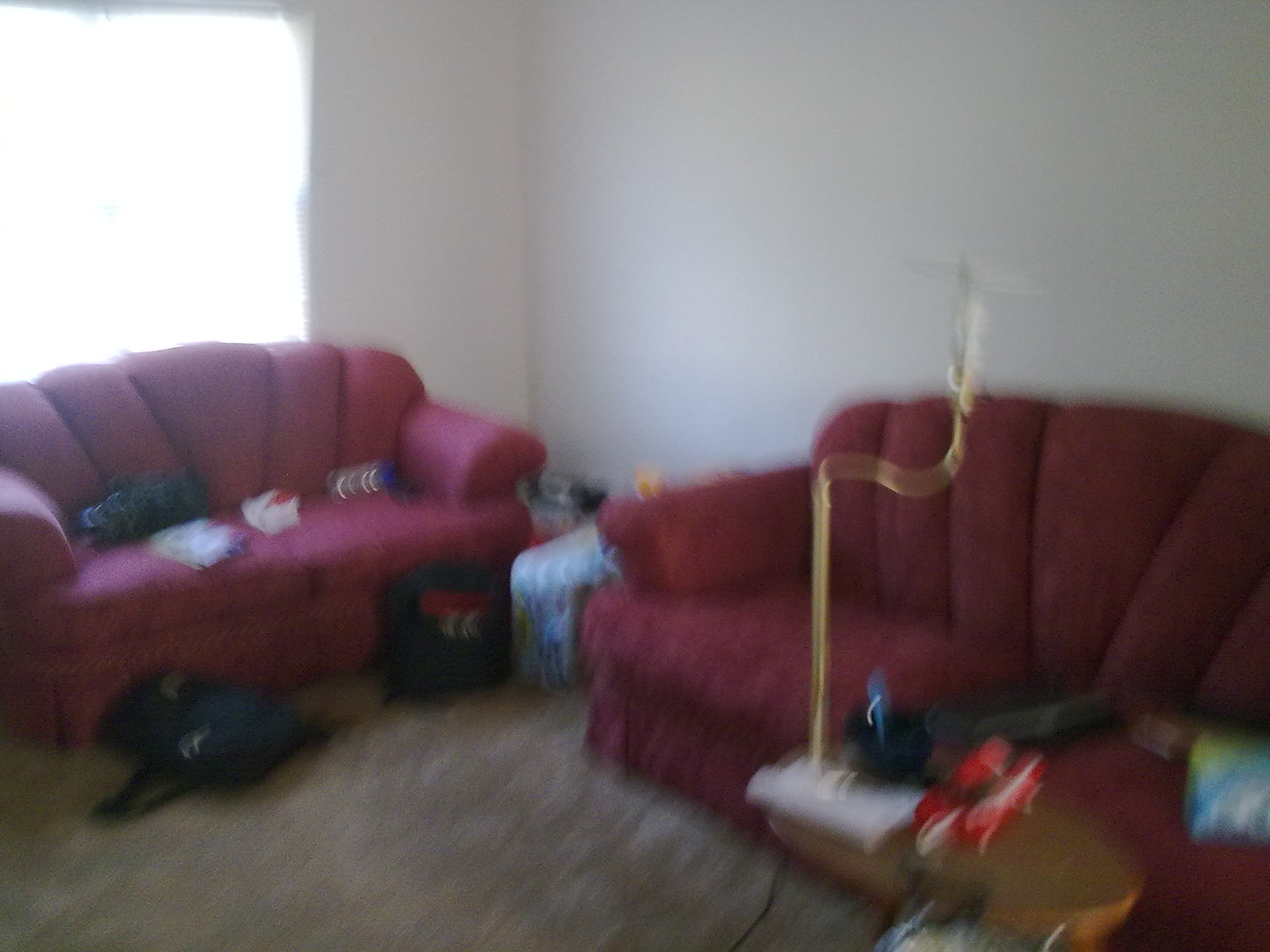A spacious yet cluttered living room is captured in an out-of-focus photograph. Various items are strewn across the room, suggesting a need for tidying. On the right side, a burgundy fabric sofa extends from the wall to the middle of the room, featuring a cloth skirt along the bottom and a back divided into long, sectioned seams. Adjacent to the sofa stands a round table adorned with a lamp composed of a white base, a straight gold metal bar that angles to the right before curving upwards. On the left side of the room, in front of a window, a matching loveseat, identical in style but smaller than the sofa, occupies the space. The overall ambiance is one of warmth and comfort, albeit in need of organization.